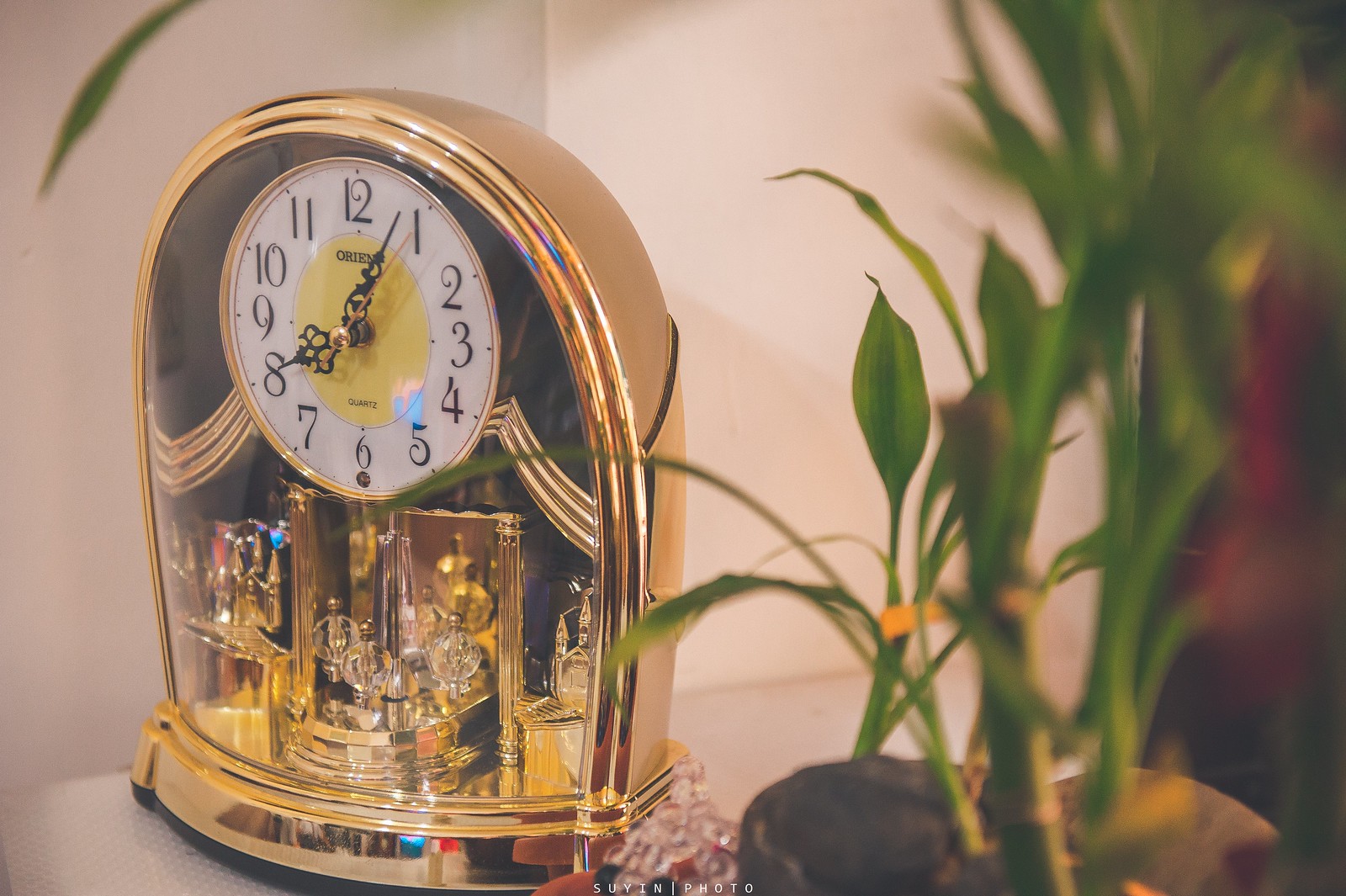The photograph showcases a decorative, gold tabletop clock set on a white surface, likely a mantle. The clock has a distinctive dome-like shape and stands on a circular base. The central clock face is white with black, ornate hands and displays the brand name "Orient" and "Quartz" in black lettering, along with a smaller yellow circle at the center. It lacks interval markings, showing only the hours 1 through 12. Beneath the clock face, there are intricate design elements including small glass bottles, crystal drops, and spherical mechanisms that sway, contributing to the clock's timekeeping. To the right of the clock, a vibrant green bamboo plant's leaves extend over part of the clock. Behind this setting, a tan wall with a hint of red can be seen, illuminated by natural lighting, suggesting it is around 8:03 a.m.